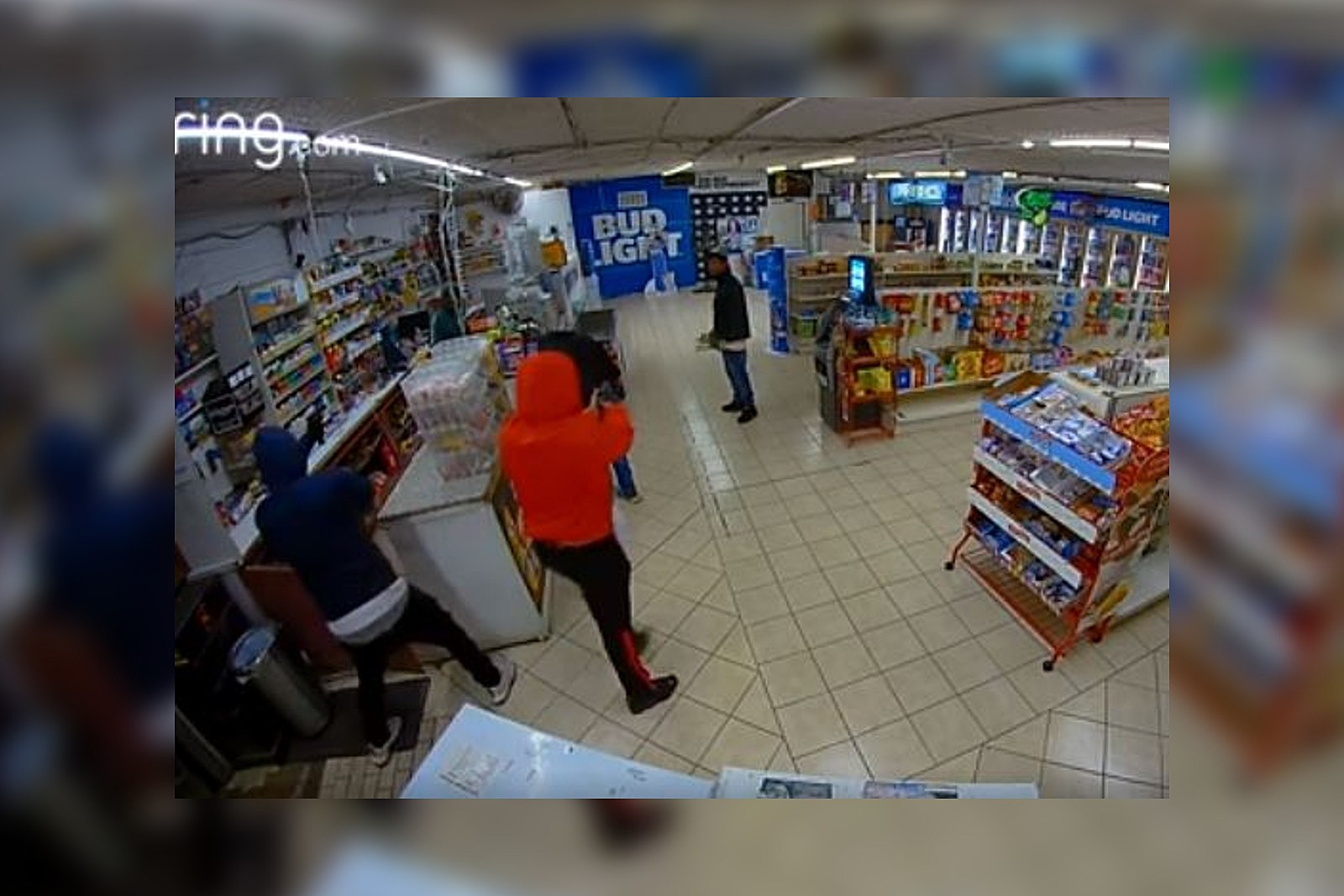A Ring camera captured this tense moment inside a convenience store, offering a glimpse into an unsettling scene. The Ring.com label, with its distinctive light blue dot above the "i," sits at the top left corner of the blurry, square-shaped background, which slightly obscures parts of the store while highlighting the main event.

In the center of the image stands a man dressed in a red sweatshirt, paired with black pants and shoes. To his left is another man in a blue sweatshirt layered over a white shirt, also donning black pants and white shoes. Both men appear to be pointing firearms, creating a threatening atmosphere.

Two customers are present in the scene. One is cowering on the counter, his head down in submission, while another waits in line, wearing a black jacket over a white shirt, blue pants, and black shoes.

The store's interior is clearly depicted with its cream-colored, tiled floor, and white ceiling adorned with bright white lights. A prominent Bud Light sign, featuring white text on a blue background, is visible at the top of the image, adding a commercial touch to the tense environment. The bright ceiling lights extend from the front of the store to the back, providing stark illumination to the unfolding drama.